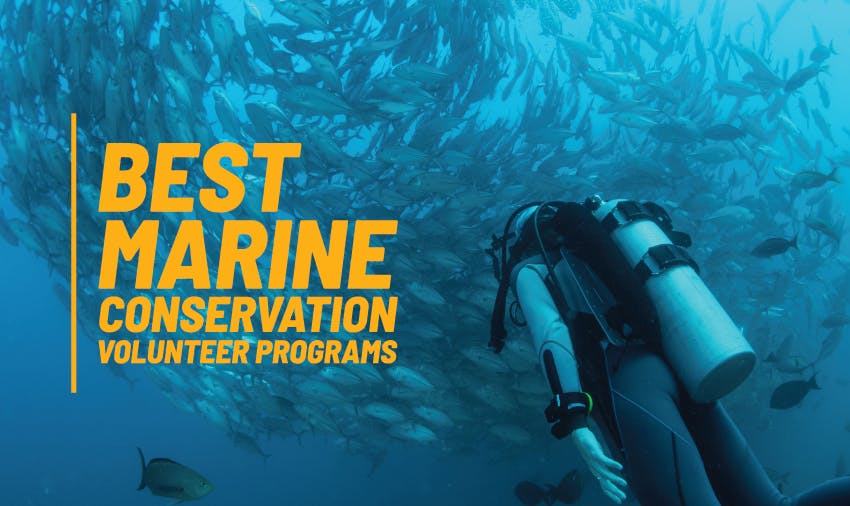The image is an underwater advertisement featuring a scuba diver positioned in the bottom right corner, looking up towards the center. The diver, clad in a wetsuit and equipped with a scuba tank, mask, gloves, and wrist equipment, is enveloped in shades of blue, reflecting the ocean's depths. Surrounding him is a mesmerizing sight of hundreds of fish swimming in a vast, swirling school that occupies most of the upper portion of the image. Amidst the school, a few darker fish stand out, and one fish notably swims towards the diver. Centrally on the left side, mustard-colored text reads, "Best Marine Conservation Volunteer Programs," adding a vibrant contrast to the deep blue hues of the scene.